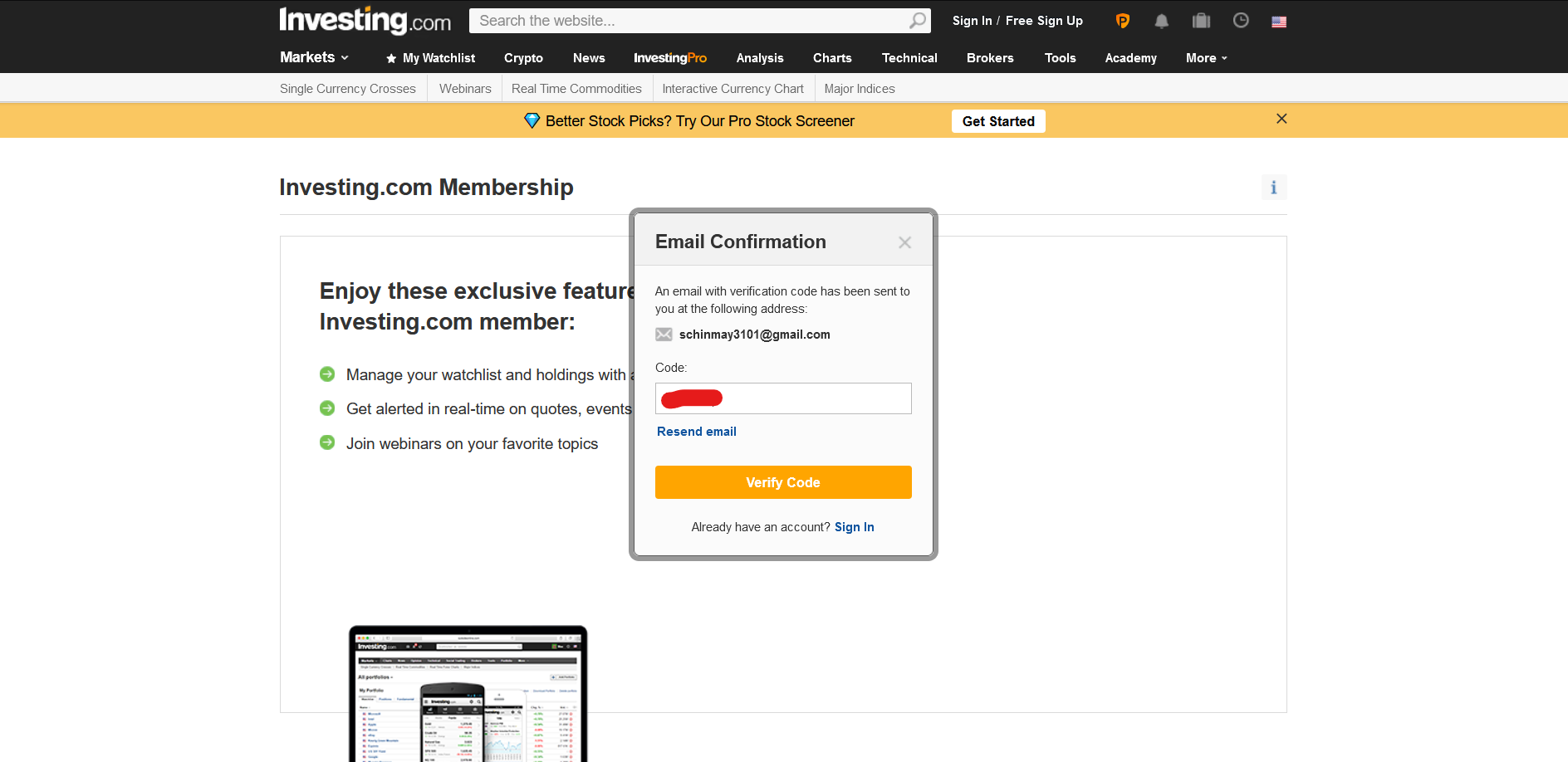This screenshot captures the interface of the Investing.com website, as viewed on a widescreen landscape format desktop or laptop. At the top, a black banner with crisp white text features the Investing.com logo to the left of the website's search bar. Adjacent to this are buttons for sign-in, free sign-up, notifications, and regional settings.

Following this, a navigation bar extends across the screen with tabs for various sections: Markets, My Watch List, Crypto, News, Investing Pro, Analysis, Charts, Technical, Brokers, Tools, Academy, and more. Immediately below this, a white banner displays options for a single currency, webinars, real-time connections, interactive currency charts, and major indices.

Highlighted in a prominent yellow banner, the site promotes its Pro Stock Screener with the message "Better Stock Picks. Try our Pro Stock Screener and get started." Underneath this is a section dedicated to Investing.com membership benefits, encouraging users to "Enjoy the exclusive features of an Investing.com member."

The subsequent area is an email verification prompt indicating that a confirmation code has been sent to the user's email address. This section includes a field for entering the code, buttons to resend the email, verify the code, and an option for users who already have an account to sign in. Below this prompt, a blue hyperlink invites users to sign in.

This detailed layout provides a comprehensive look at the Investing.com homepage, showcasing the various features and user prompts available on the site.